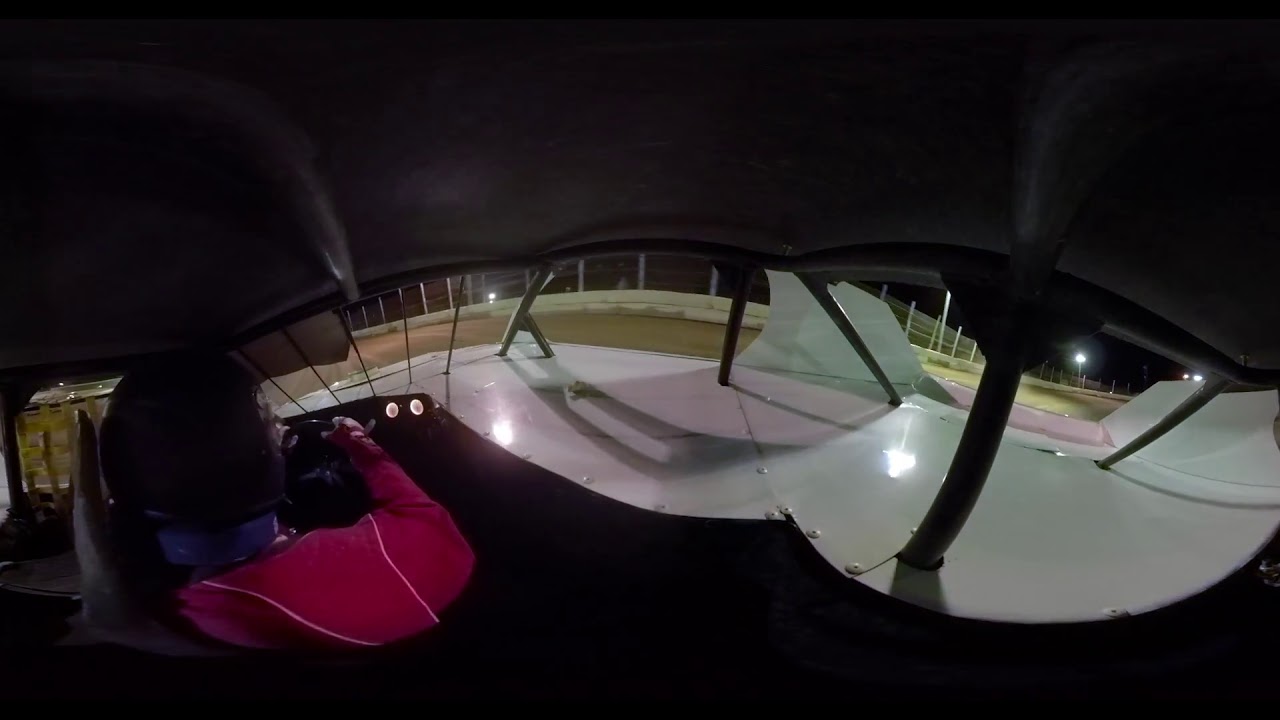This is a photograph taken with a fisheye lens, capturing the interior of a white metal vehicle, possibly a small prop plane or some kind of off-road vehicle, at night. The image shows a person sitting on the far left side, wearing a black helmet and a red jacket or long sleeve shirt, holding onto a steering wheel. The vehicle features several white metallic panels bolted together and an opening or window through which the driver sees out. Various screens and dials are visible on the panel in front of the driver. The vehicle is situated on a dirt track with high fencing and wall barriers surrounding it, and the dark night sky is illuminated by lights mounted on poles.